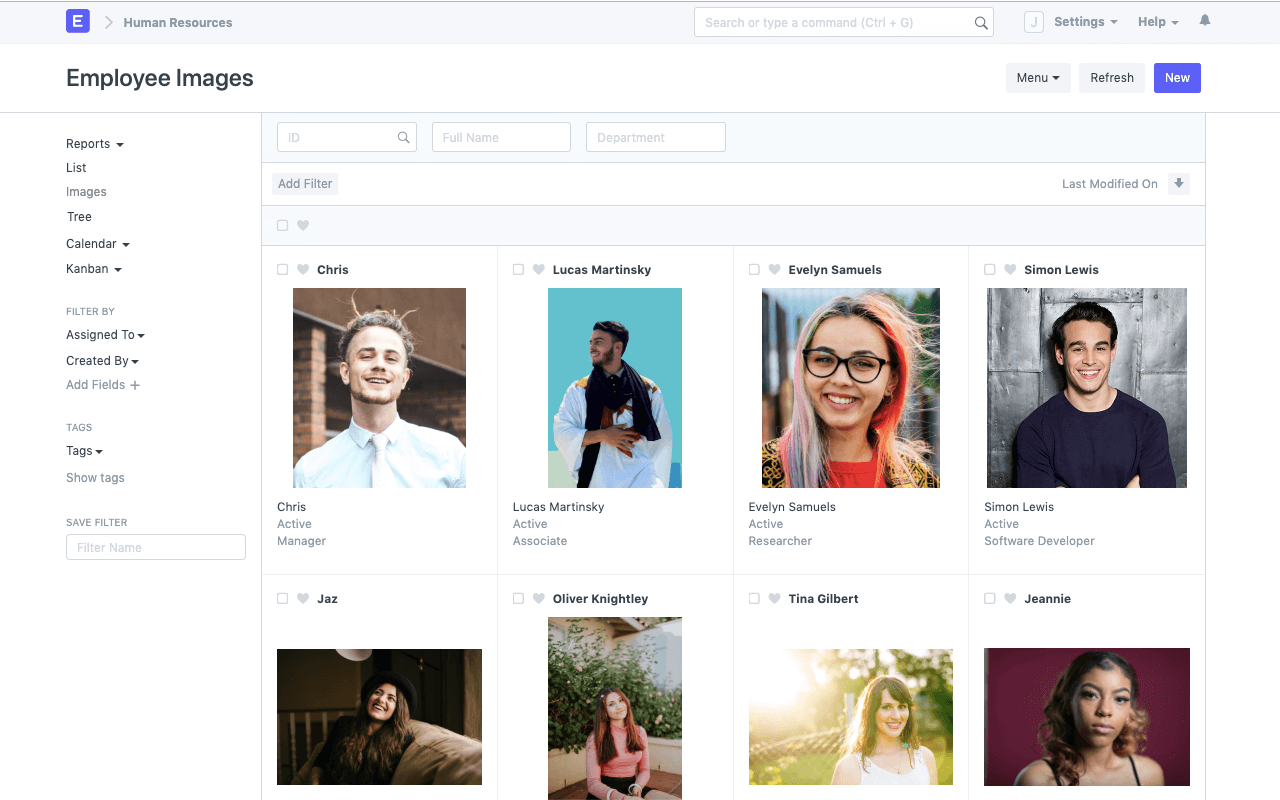The image displays a company's human resources interface, featuring a Periwinkle icon with the letter "E" in a square positioned at the top, accompanied by the label "Human Resources." Directly below this, there is an "Employee Images" section. On the left-hand side of the interface, a vertical menu offers various filtering options, including "List Images," "Tree," "Calendar," and "Kanban." Additional filters allow sorting by "Assigned To," "Created By," or customized fields, with the possibility of adding tags and saving filters with specific names. This setup appears to facilitate efficient filtering of employees within the company.

Shown in the image are eight employees, each represented by a casual yet professional headshot that conveys a natural and personal vibe. The employees listed include:

- Chris, identified as a manager
- Lucas Martinsky, noted as an associate
- Evelyn Samuels, marked as a researcher
- Simon Lewis, labeled as a software developer
- Jazz
- Oliver Knightley
- Tina Gilbert
- Jenny

Unfortunately, the detailed information for the last four employees is not visible in the bottom section of the image. The overall impression suggests this interface is part of a human resources program designed to manage and filter both active and inactive employees based on various attributes such as their reporting structure or the creator of their listing in the HR directory.